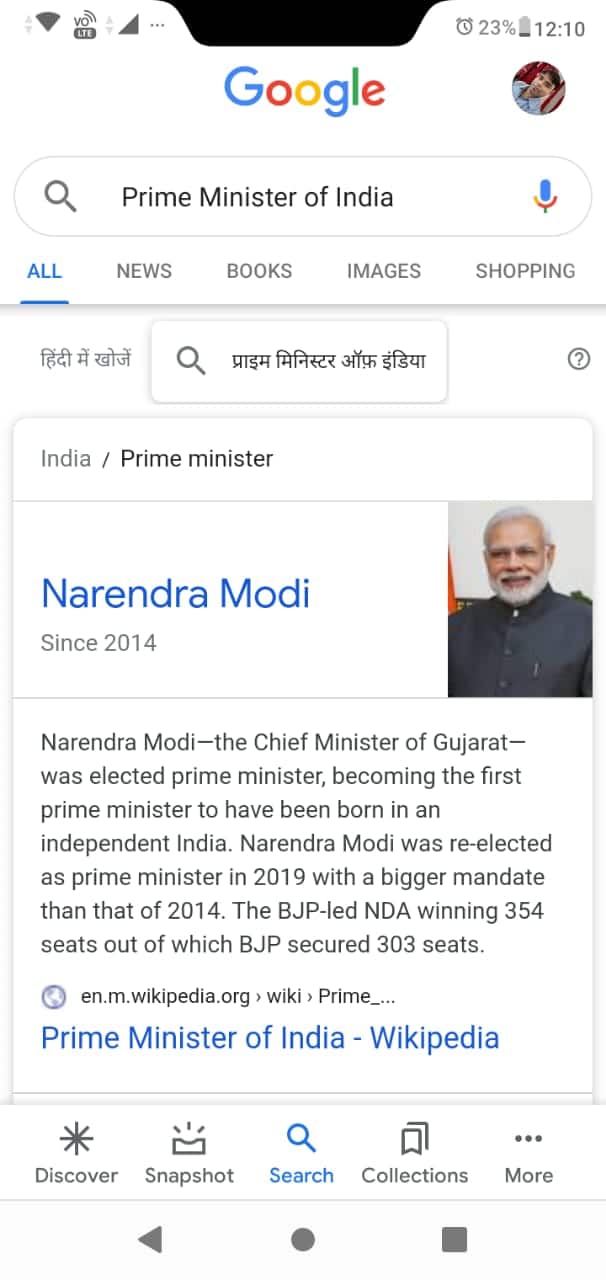The image captures the results page of a Google search. At the top of the page, system icons such as battery percentage, a clock, and signal indicators are visible. Prominently displayed on the page is the Google logo, featuring its iconic blue, red, yellow, and green colors. In the search bar, the query "Prime Minister of India" is entered, accompanied by a colorful microphone icon on one side.

Below the search bar are various navigation tabs including "All," "News," "Books," "Images," and "Shopping." Additionally, the interface offers a search option in the Indian language. The search results reveal an informational snippet about the current Prime Minister of India, Narendra Modi, who has held the position since 2014. The text highlights that Narendra Modi, formerly the Chief Minister of Gujarat, was elected as Prime Minister, becoming the first to be born in an independent India. It further mentions his re-election in 2019 with a stronger mandate, where the BJP-led NDA won 354 seats, with BJP securing 303 of those.

A hyperlink to the Wikipedia page titled "Prime Minister of India" is clearly marked in blue. At the very bottom of the screen, various navigation options such as "Discover," "Snapshot," "Search," "Collections," and "Books" are displayed, providing users with additional functionalities to enhance their search experience.